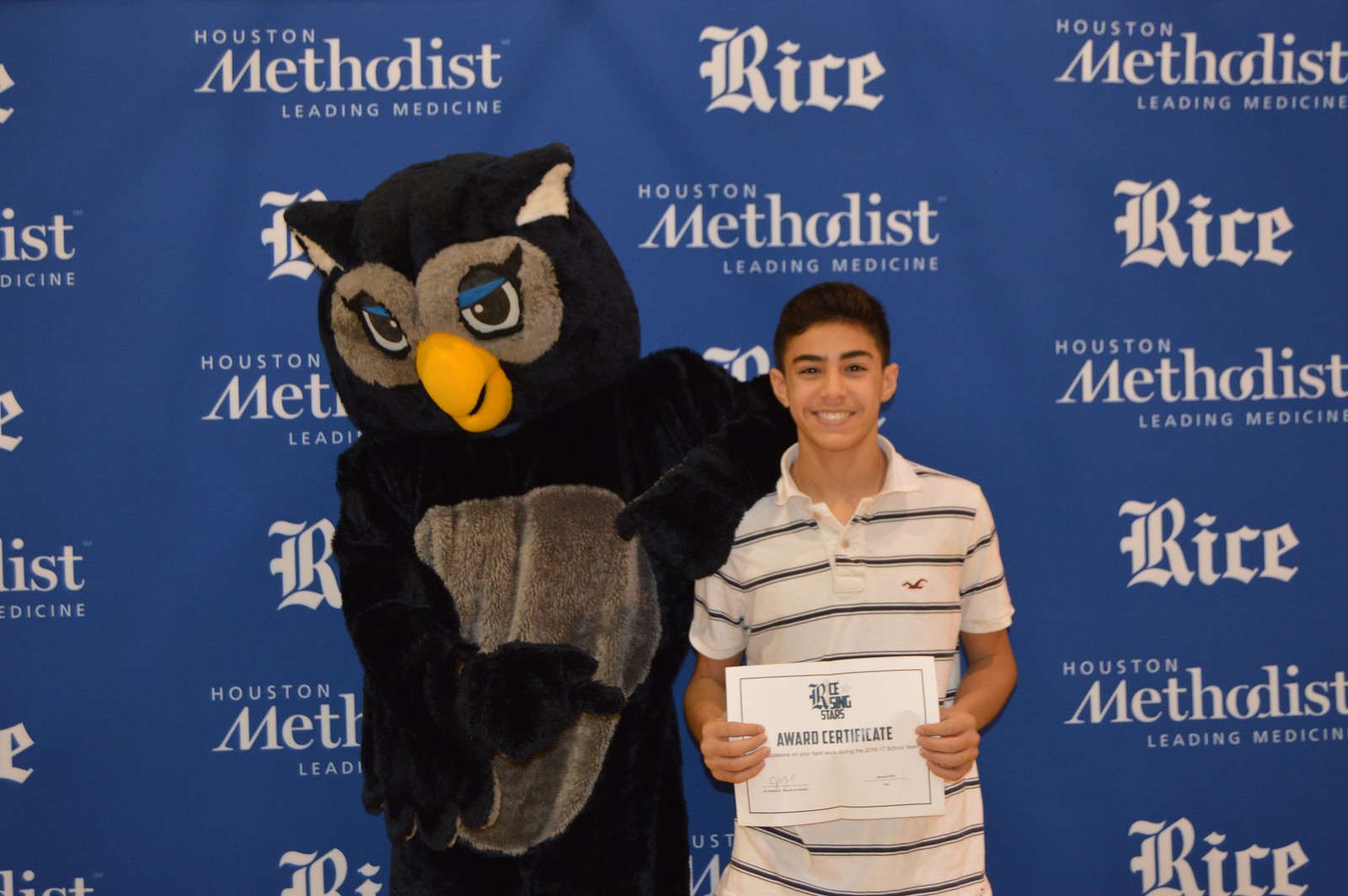The photograph features a smiling young Latino boy with dark hair and brown eyes, standing proudly while holding an award certificate. He is dressed in a cream striped shirt with horizontal dark bars. To his left stands a person in a detailed owl costume, featuring a dark body, gray belly, yellow beak, white ears, and blue eyelashes above their dark eyes that are encircled in white. The background is a blue fabric banner adorned with repeating white logos alternating between "Rice" in a gothic script and "Houston Methodist Leading Medicine." The boy, standing close to the owl mascot, looks directly at the camera, exuding happiness and pride.